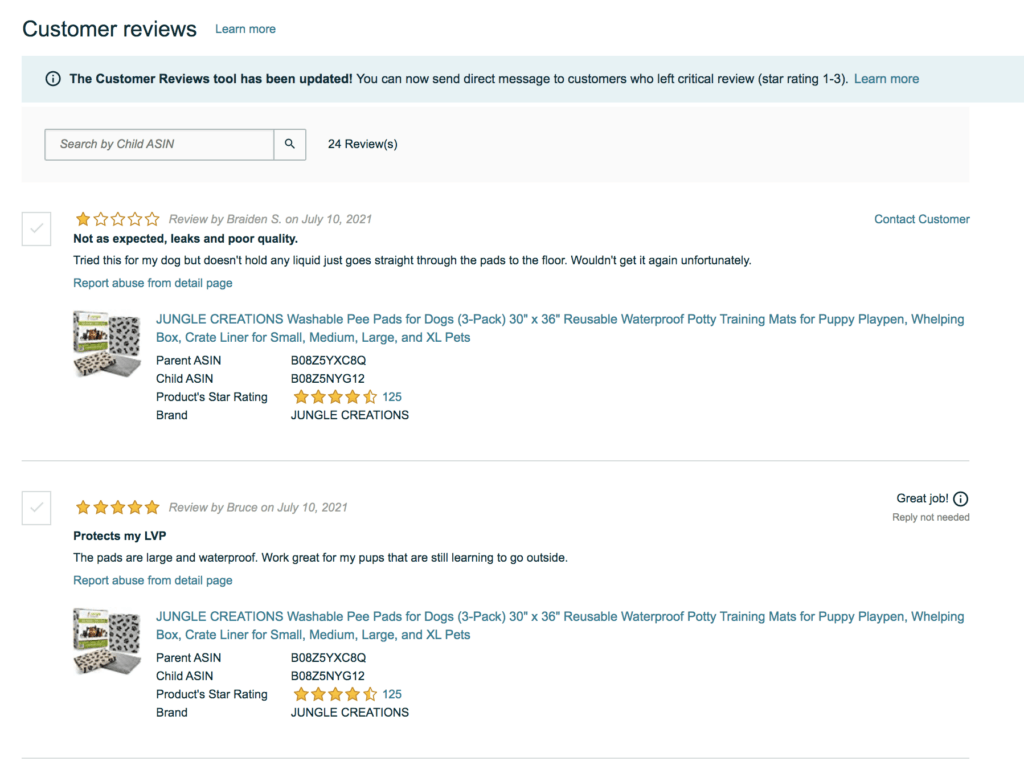The image displays a review page on Amazon's website. At the top left corner, it prominently reads "Customer Reviews" in black font. Adjacent to this on the right, a link marked "Learn More" appears in small blue text, signifying it's clickable due to its distinct color. Below this section, a noticeable light blue banner houses a dark blue circular icon with an eyeball graphic, symbolizing informational content. The banner exclaims in bold blue lettering, "The Customer Reviews Tools have been updated!" Following this, in the same blue hue but non-bold, it informs users, "You can now send direct messages to customers who left critical reviews (Star Rating 1-3)." Another "Learn More" clickable link appears here in a slightly lighter blue font.

Beneath this banner, a light gray section features a search bar outlined in gray. On the right side of the bar, a small square with an angled magnifying glass icon appears, with "Search by Child ASIN" written in italicized gray font inside. To the right of this search bar, in bold black text, it shows "24 Review(s)."

Below this, the page presents two reviews. Each review has a light gray tick box on the left, marked with light gray check marks. The first review displays a one-star rating, indicated by one filled orange star followed by four outlined stars.